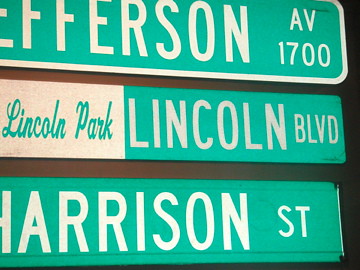The photograph portrays a collection of street signs displayed against a dark background, possibly a table or wall, suggesting the setting is indoors. The primary focus of the image is on three street signs, all uniformly green with white, sans-serif lettering. 

The topmost sign reads "JEFFERSON AV 1700", though the first letter is cut off, making it appear as "EFFERSON AV 1700". Below it, a sign in a different style and size indicates "LINCOLN PARK" in script lettering on a white background, followed by "LINCOLN BOULEVARD" on a green background, segmented into two distinct sections. The next sign reads "HARRISON STREET", although the initial "H" is partially out of the frame.

Of particular note is the design consistency: the "JEFFERSON AV" sign features a white border, unlike the other signs which lack borders. The careful arrangement and clear visibility of each sign against the contrasting black background emphasize their details and lettering styles, providing a study in the visual and functional aspects of street signage.